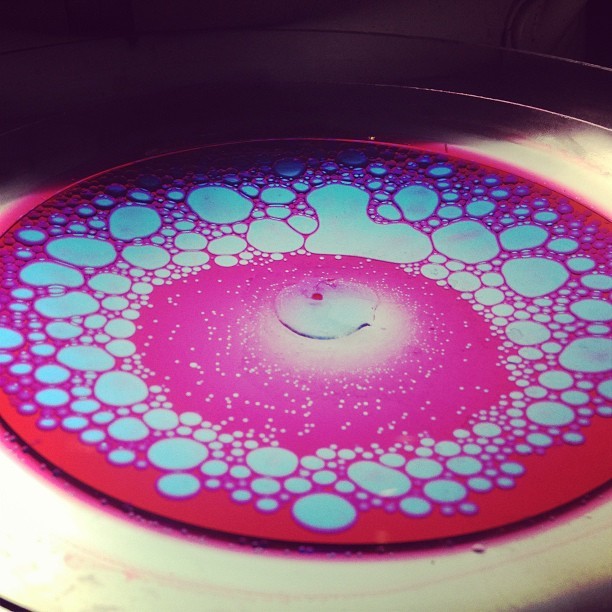This color photograph features an enigmatic liquid art piece presented in a circular shape. The top section of the image is engulfed in dark black, creating a stark contrast with the vibrant, radiant colors below. At the heart of the circle, a mesmerizing combination of pink and red hues dominates, resembling a liquid medium that remains distinct and unmixed. Scattered throughout this central area are various drops of light blue liquid, each outlined by a subtle purple hue, evoking the mesmerizing effect of oil and water interaction. At the very core of the circle lies a bright white element, possibly a reflection off a glass-like surface, marked with a conspicuous red dot in its exact center. This vivid arrangement is framed by a prominent white outer circle, encapsulating the entire artistic composition.